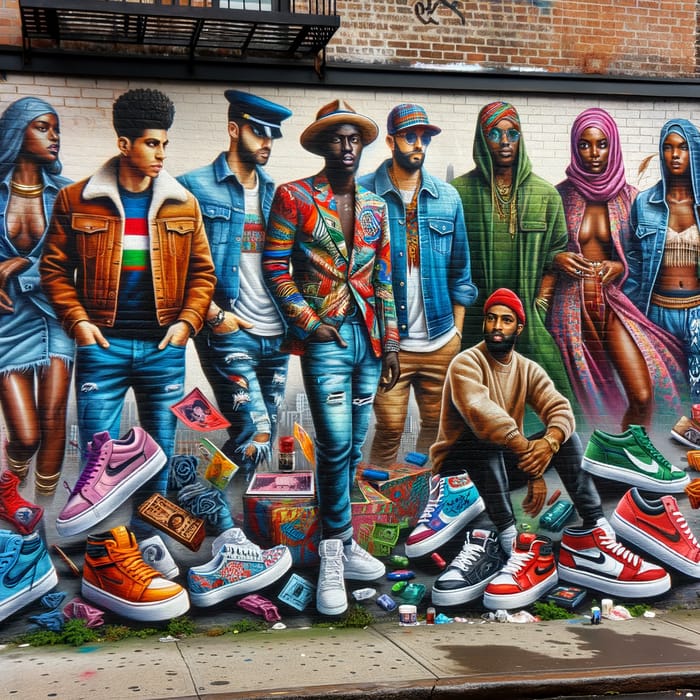The mural depicts a vivid and diverse collection of roughly 10 African-American figures, both men and women, standing together against a white backdrop with a red brick building at the top. Starting from the far right, a woman adorned in a blue headdress and a light cream-colored bra that exposes her chest and upper stomach, including a black hole for a belly button, stands prominently. Next to her is a woman in a pink headdress and an open pink and purple robe, revealing the sides of her breasts, and her hand gracefully placed in front of her stomach. Adjacent to her is a woman in a green robe with blue sunglasses. Beside her, a man in a blue denim jacket, white shirt, brown pants, and a blue hat stands confidently. Another man nearby dons a fedora, a colorful vest with splashes of red and green, and distressed blue jeans. Following him, a man in a blue policeman-like hat and denim jacket with his hands in his pockets adds to the lively mix. Another man sporting a large afro, a brown jacket with a red undershirt, and striped blue jeans stands to the left. Finally, a woman on the far left is draped in a denim-colored wrap with a blue headdress, revealing her breasts from the front.

At the bottom of the mural, a man with a red beanie, brown sweatshirt, black pants, and a gold watch is seated cross-legged, surrounded by a striking array of Nike tennis shoes in various colors and designs—green, red, red and white, black, blue with a black signature, and one with a floral design on a white sole. The sidewalk beneath them is speckled with watercolor dots and a touch of moisture, adding a dynamic texture to the scene.